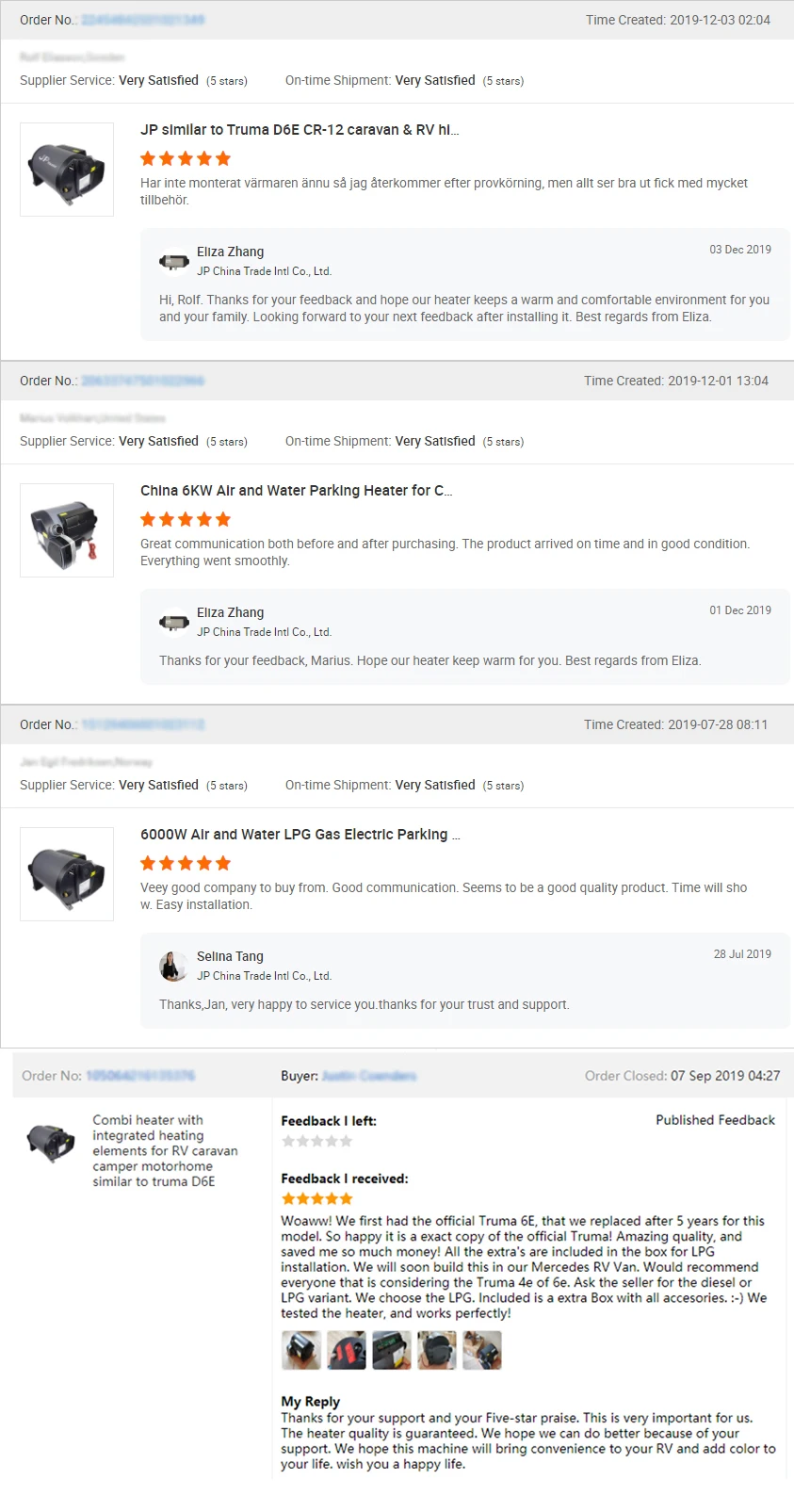### Detailed Caption for the Image:

The image displays a webpage interface where users can leave and view reviews. The top portion of the page shows several customer reviews, encased in a black border. On the left-hand side of the page, the term "Order Number" is prominently printed in black text, though the actual order numbers are blurred out. These numbers originally appear in blue.

To the right, in black text, there's an entry that reads: "Tom created...2019-12-03," followed by "02-1.04." The username and site name are also present but have been blocked out.

The first review featured is written in a non-English language. It mentions that the supplier service is "very satisfied" with a rating of five stars, as is the on-time shipment. Additionally, the reviewer identifies the item as "JP similar to Truma D6-ECR-12, cameraman in RV at high..." and gives it five stars. The response from the supplier, a person named Eliza, reads: "Hi, Rolf, thanks for your feedback. I hope our heater keeps a warm and comfortable environment for you and your family. Looking forward to your next feedback after it's done. Best regards, Eliza."

The second review on the page, also attributed to a user named Tom, is shown with the date "2019-12-01-13-04." This review states that the supplier service was "very satisfied" and gave it five stars, along with the on-time shipment. The reviewer praises the "great communication, both before and after purchasing the product," noting that the transaction had "reliable timing" and went smoothly. This review is also replied to by Eliza, saying: "Thanks for the feedback, Marius. Hope our heater keeps warm for you. Best regards, Eliza."

The overall layout of the page is simplistic and functional, focusing on displaying user reviews, ratings, and supplier responses prominently.